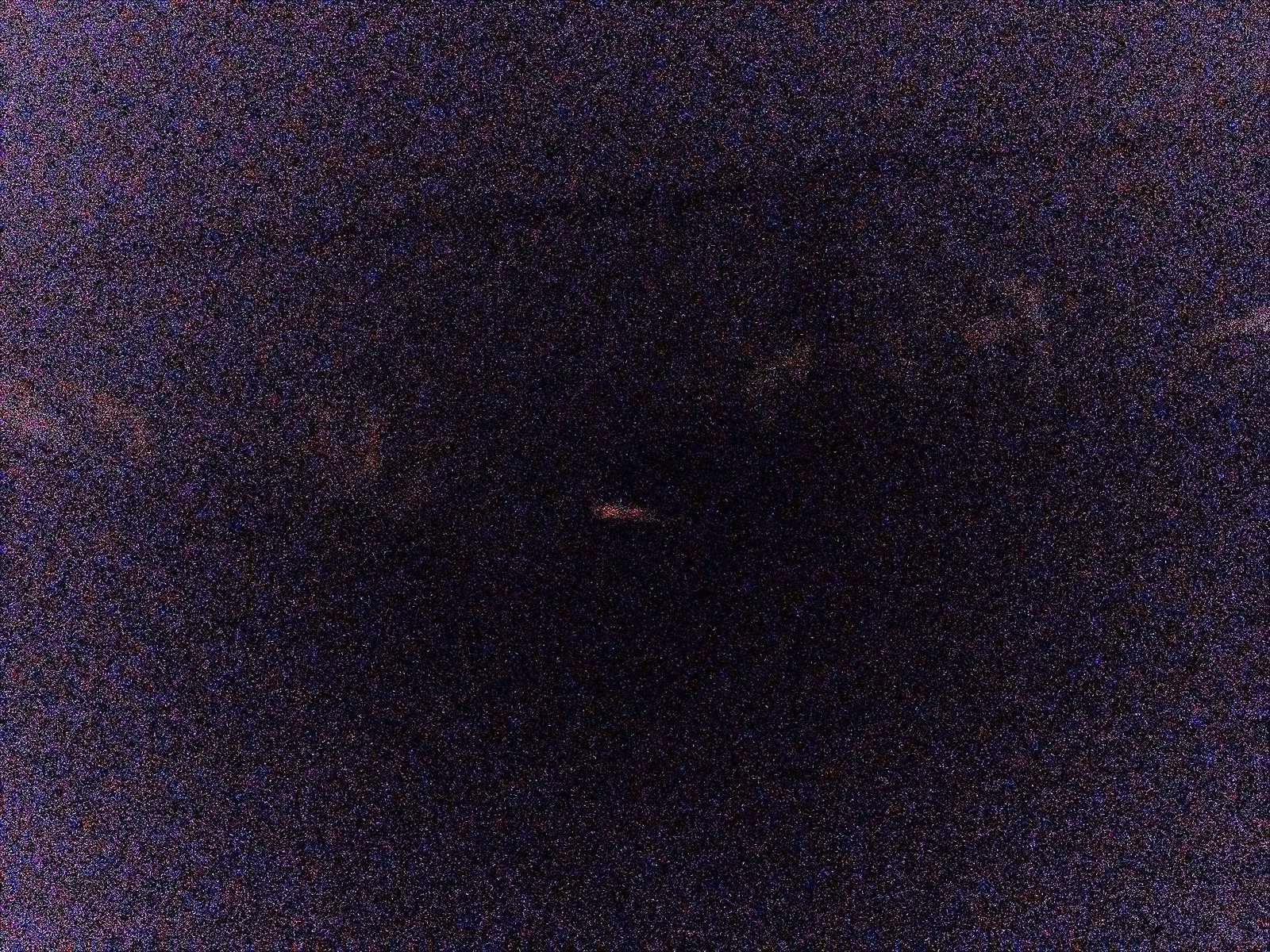A grainy and heavily blurred photograph dominated by a dark pink hue, interspersed with hints of blue. The image appears as if taken through a frost-covered window or windshield, obscuring any discernible features. Five or six brighter, orange spots punctuate the center, surrounded by a contrasting blackish area, adding a sense of depth and mystery to the otherwise abstract composition.